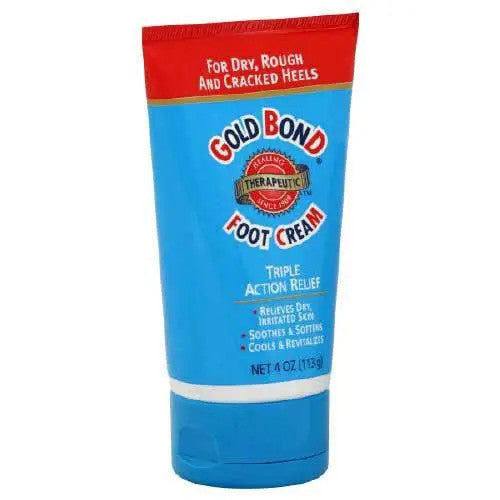The image depicts a tube of Gold Bond Foot Cream, standing upright on its blue flip-top cap. The main body of the tube is light blue, with a darker blue cap and a small red section at the base. The text on the tube indicates that the product is designed for dry, rough, and cracked heels, promising "Triple Action Relief" that relieves dry, irritated skin, soothes and softens, and cools and revitalizes. Prominently displayed beneath the Gold Bond logo is a red, circular "therapeutic" emblem. The tube also specifies that it contains 4 ounces (113 grams) of cream. There is a noticeable white neck around the top part of the cap, and the image is slightly blurred, making the precise founding date of the brand difficult to read.